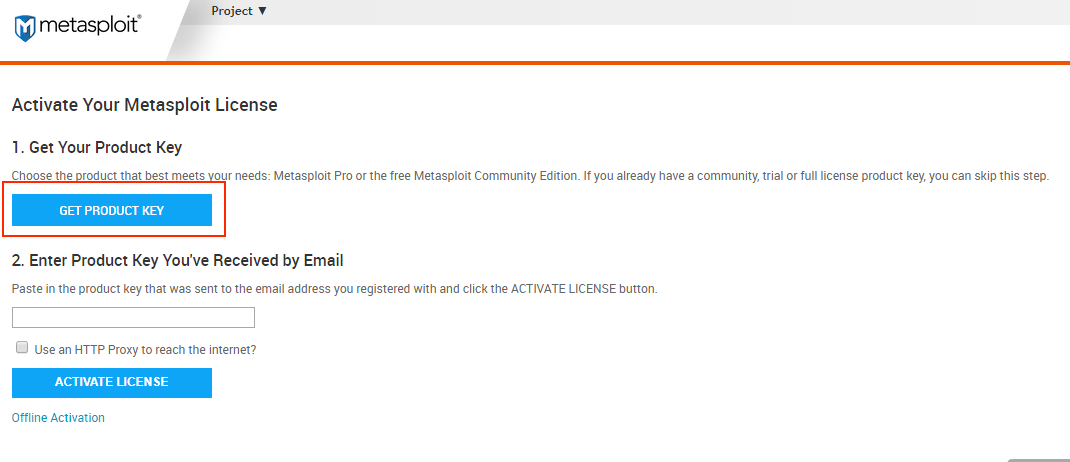Category: Websites

At the very top of the page, a white 'M' is prominently displayed against a blue background, adjacent to the word "Metasploit." Directly below, the word "Project" appears with an arrow pointing downward, accompanied by an orange line underneath.

The main section starts with a bold heading: "Activate Your Metasploit License." The instructions continue, guiding users to obtain their product key with options to choose between "Metasploit Pro" and the complimentary "Metasploit Community Edition." It notes that users with an existing community trial or full license product key can bypass this step.

A red outline highlights a blue box labeled "Get Product Key." Below, the instructions prompt users to enter the product key they've received via email, asking them to paste it into the provided field and click the "Activate License" button.

Additionally, users have the option to check a box labeled "Use an HTTP proxy to reach the internet?" Below this, a blue box with white letters provides the button for "Activate License." Finally, near the bottom of the page, there is a clickable link for "Offline Activation."